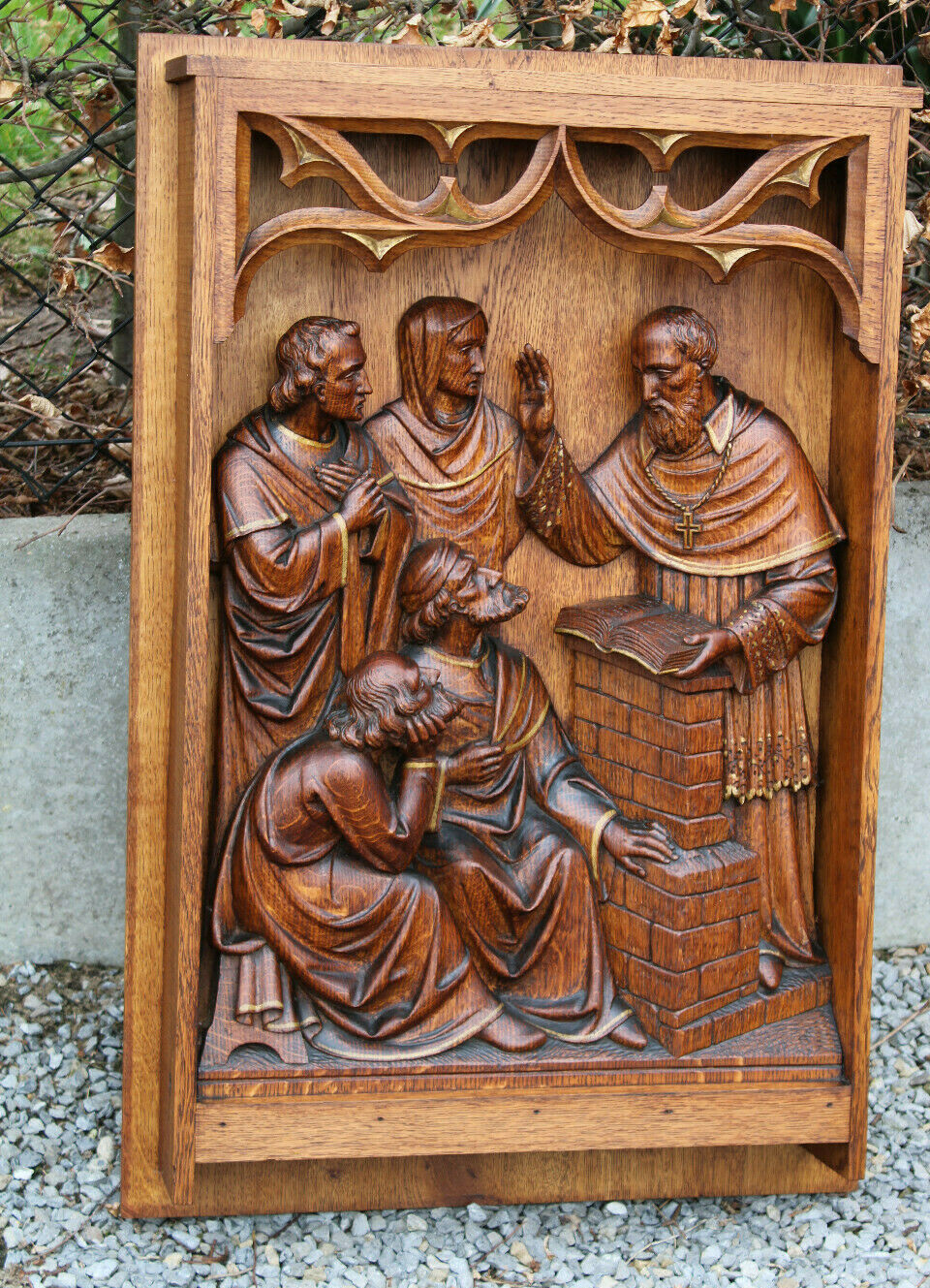This photograph captures a beautifully intricate wooden sculpture depicting a scene involving a total of five figures. At the center, a priest is prominently featured, identifiable by a cross necklace around his neck. He stands behind a small, brick-like podium, or perhaps an altar, upon which an open book, likely a Bible, rests. The priest's right arm is raised, possibly in a gesture of blessing or preaching.

The scene is framed within a tall, rectangular wooden area with a deep inset and is crowned by a subtle archway at the top. The other four figures are arranged in front of the priest, with two standing and two seated. The detailed carving showcases a historical or biblical context, enhanced by the priest's traditional attire.

The craftsmanship highlights the artist's skill, as the wood features a range of brown, beige, and blonde hues. The entire sculpture rests outdoors on a rocky, pebbly surface and is positioned against a chain-link fence, presenting a stark contrast between the refined artistry and its rugged setting.